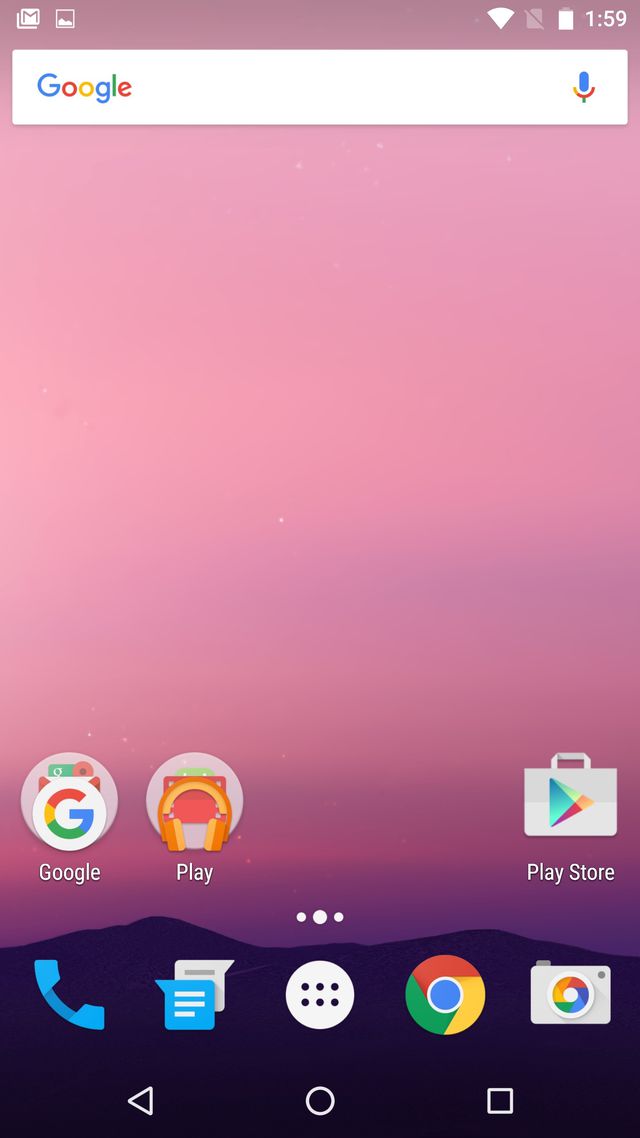This image, captured on a smartphone, presents a stunning twilight sky transitioning from a pink hue at the top to a rich purple closer to the horizon. The silhouette of distant hills forms a very dark purple against the blackened foreground, adding depth to the serene landscape. 

At the upper left corner of the screen, several on-screen icons are visible: a white rectangle with a male icon on top, followed by an image icon. Adjacent to these is a fan-shaped symbol in white, a rectangle intersected by a line, and the battery icon indicating a high charge. The time displayed is 1:59. Centrally positioned on the screen is a white rectangle with the Google logo to the left and a microphone icon to the right.

Below this main section, the home screen icons are partially visible. The most prominent is the Google logo, flanked by faintlessly overlapping icons within a circular pink gradient. To its right, there is a stack of icons, with orange headphones at the front, labeled "Play." Further to the right, the Google Play Store icon—a shopping bag with a triangular play symbol—stands clearly labeled "Play Store."